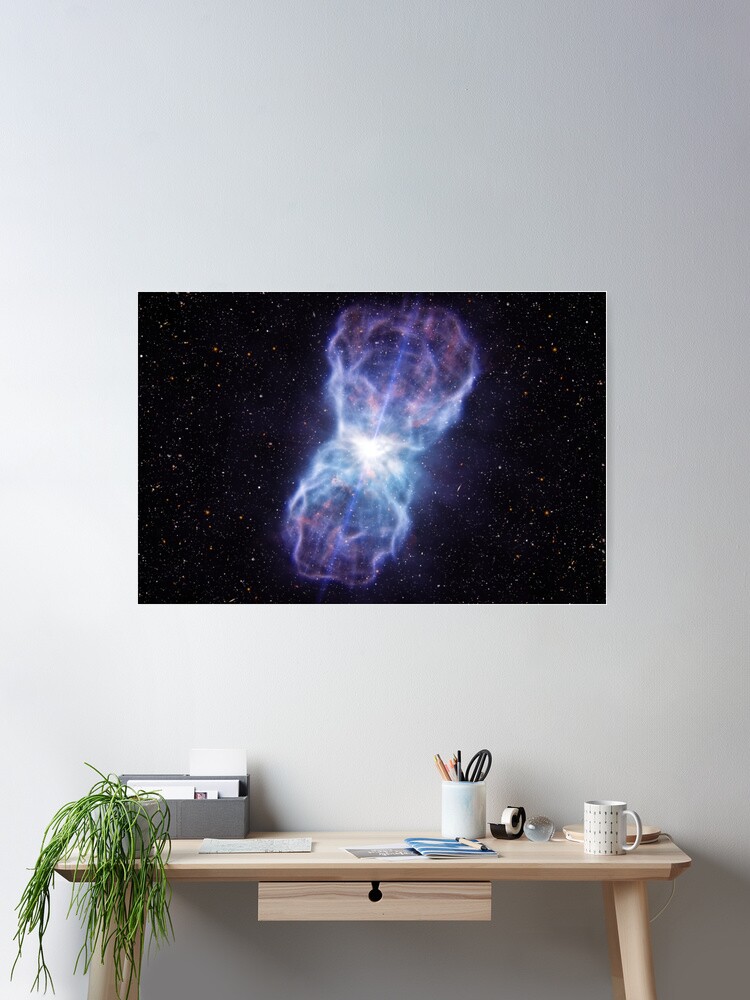This color photograph captures the inside of a home office area. A white wall serves as the backdrop for a striking piece of artwork above a light wood-colored desk. The artwork depicts a vivid outer space scene, characterized by a starry black sky and a supernova in the center, emitting beams of plasma upwards and downwards. The nebula within the photograph consists of electric blues, purples, pinks, and whites, arranged in an explosion pattern that reveals a celestial body, possibly a star, with a bright, central light.

Below the artwork, the light tan desk features a single central drawer with a keyhole-like finger pull. The desk is adorned with various objects: on the left-hand corner is a hanging plant, its green leaves gracefully drooping down. Adjacent to it is a gray desk organizer containing envelopes and papers. A cup holding pencils and scissors, a black tape dispenser, and some scattered papers are present as well. A small white coffee mug with a pattern and a crystal ball also occupy the desk space. To the right, a white adjustable desk lamp illuminates the scene, completing the organized yet somewhat cluttered workspace.